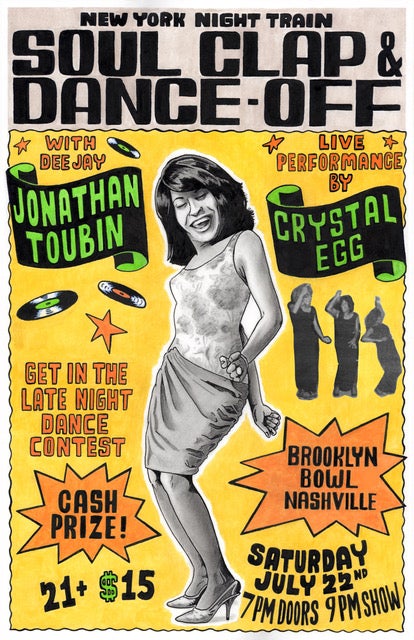The image is a vibrant nightclub flyer designed in a comic book style, measuring approximately five inches tall by three inches wide with a thin, nearly transparent white border. At the top, against a light pinkish or tan background, bold black print reads "New York Night Train Soul Clap and Dance Off," with "New York Night Train" appearing in smaller text than the rest of the title. The majority of the flyer features a bright yellow background structured into two columns of text and images on the left and right edges. 

Dominating the center is a black-and-white photograph of a young woman with long black hair, eyes closed, dancing spiritedly in a sleeveless, tight gray dress that reaches her knees, paired with high heels. She epitomizes the energy of the event.

On the left side of the flyer, text announces DJ Jonathan Toobin and a call to action for the late-night dance contest, highlighting a cash prize with an orange starburst around the text "$21 plus $15." On the right side, details about a live performance by Crystal Egg are prominent, including an image of the three performers and mentions of Brooklyn, Bowl, and Nashville.

The flyer concludes with essential event details: "Saturday, July 22nd, 7 p.m. doors, 9 p.m. show," ensuring all vital information about the time, location, and activities is clear.